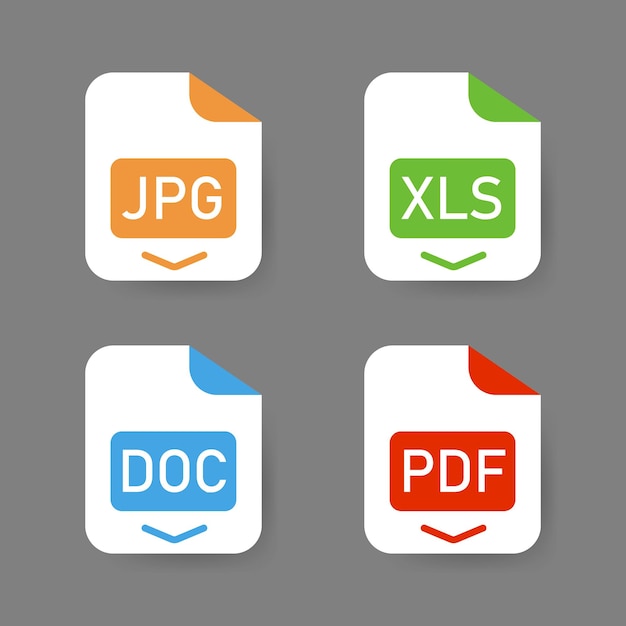The image presents a square format set against a gray background, featuring four simplistic computer folder icons arranged in a 2x2 grid. Each icon is depicted as a rounded white rectangle with a folded top-right corner, known as a "dog ear," which is color-coded to indicate different file types. The top-left icon represents a JPG file, characterized by its orange dog ear and text box. Adjacent to it on the top-right is an XLS file, distinguished by green. On the bottom row, the left icon signifies a DOC file with blue accents, and the right icon indicates a PDF file with red features. All icons have their respective file type text displayed in white letters against their colored backgrounds, creating a clear and organized visual representation of different document formats.